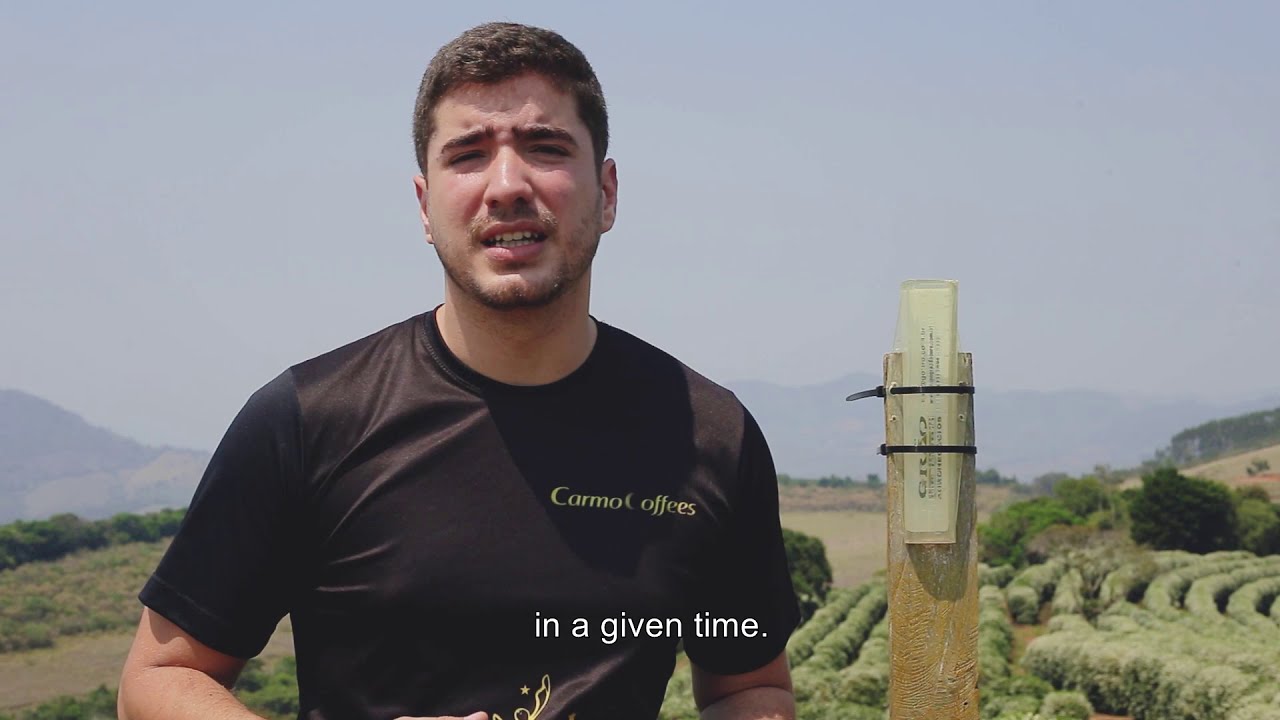The image captures a young man standing outdoors under a vibrant blue sky, with a backdrop of hazy mountains and rolling brown hills adorned with rows of green vegetation, resembling a garden or farm. In the foreground, the man is positioned slightly to the left of a wooden post that has a piece of paper zip-tied to it, likely serving as a marker for the plants nearby. He has short, dark brown hair, nearly black, and a light stubble on his face. His black t-shirt bears the words "Carmo Coffees" in yellow font, suggesting a connection to coffee farming. His expression is open-mouthed, showing his teeth as if mid-sentence, with his eyes squinting, possibly due to the sun. The overall scene indicates a lush and industrious agricultural setting.